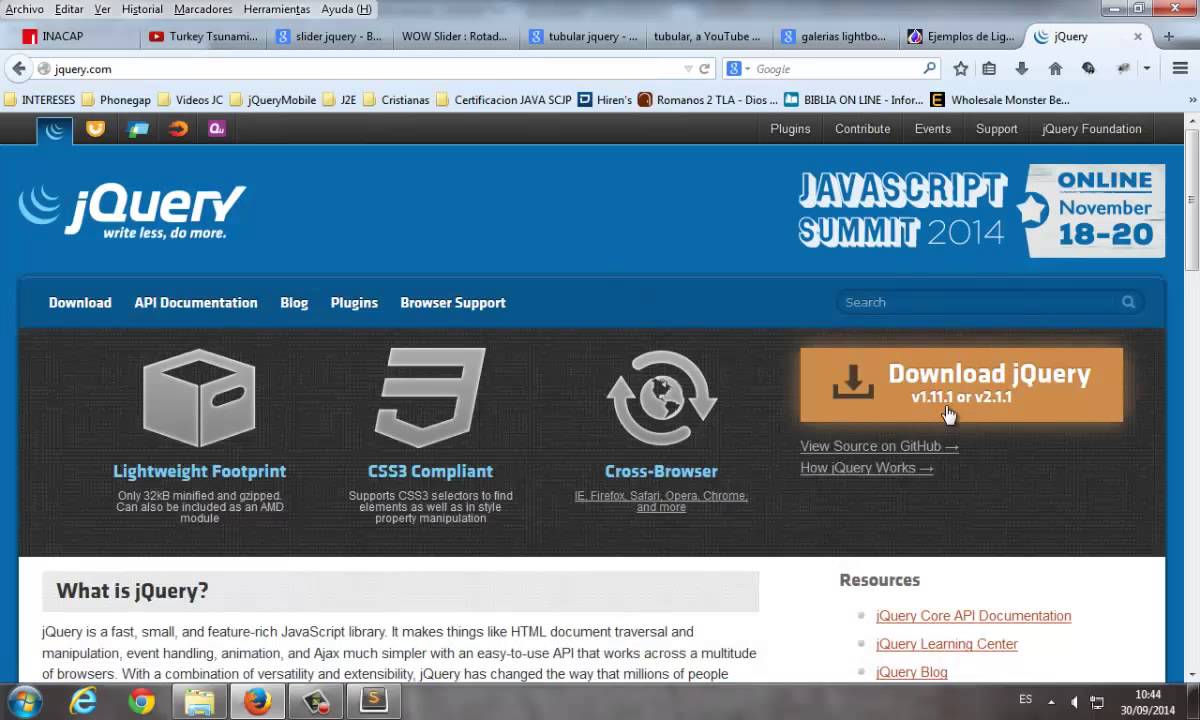The image showcases an open web browser window with approximately nine tabs, although the content of these tabs is indiscernible due to the blurriness. The address bar clearly displays "jQuery.com." Just below the address bar is a black border featuring menu options, including "Plugin," "Contribute," "Events," "Support," and "jQuery Foundation." 

The main section of the page has a blue background prominently displaying the jQuery logo and the tagline, "Write Less, Do More." On the right side, there is text advertising the "JavaScript Summit 2014," held online from November 18-20. Below this advertisement, additional navigational links are listed, such as "Download," "API Documentation," "Blog," "Plugin," and "Browser Support."

A search box is visible, underneath which there is another black box containing buzzwords and feature highlights like "Lightweight Footprint," "CSS3 Compliant," and "Cross Browser."